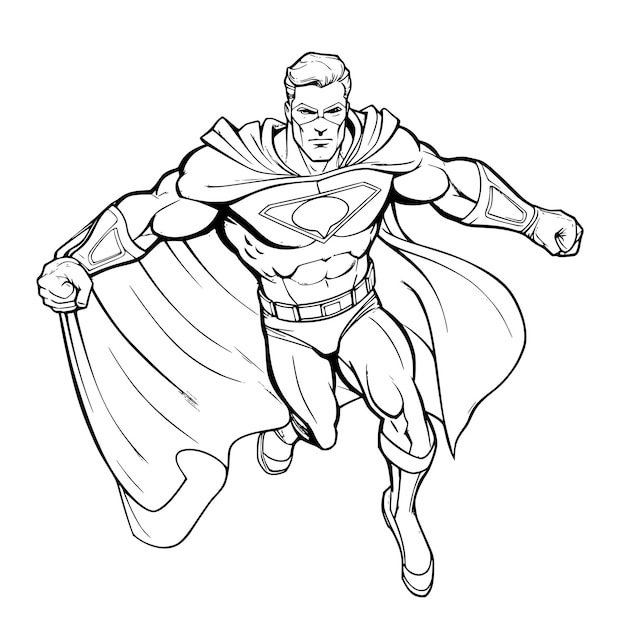This is an artist's rendering of a muscular, black-and-white superhero positioned centrally against a white background. The superhero is depicted with a large, flowing cape and a distinctive symbol on his chest, resembling a diamond without the classic 'S' of Superman. He is wearing a mask covering his eyes, exhibiting a heroic stance with both arms extended at his sides. His detailed physique includes abs, wrist guards, and boots, complemented by a belt and a jock with a belt buckle. The short, blonde hair is visible, adding to the character's strong and determined appearance. One leg appears to be stepping forward, and part of his cape is drawn slightly with the movement of his left hand. There is no text or additional objects in the image, emphasizing the dramatic and powerful portrayal of the superhero.